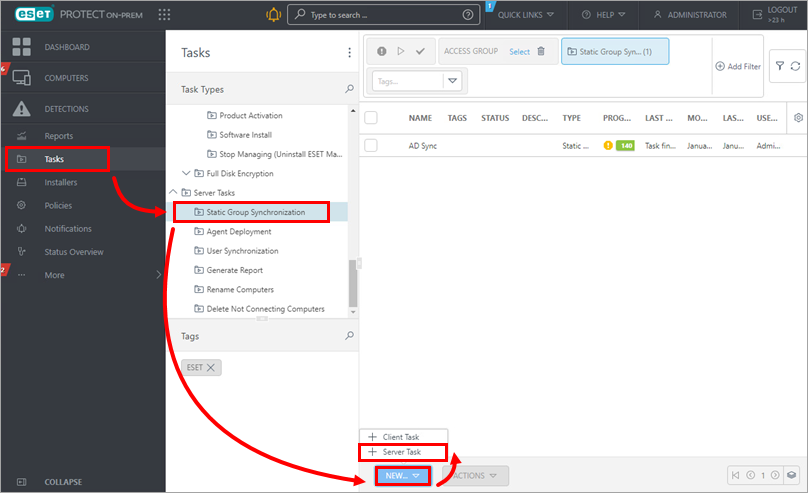This is a detailed screenshot of the dashboard or account page of the ESET PROTECT software. The interface features a dark gray vertical sidebar on the left and a dark gray horizontal bar across the top. In the top-left corner, the ESET logo is prominent in white and green, followed by the word "PROTECT" in uppercase letters next to the logo. Adjacent to this, there is a grid button, and to its right is a yellow bell icon for notifications. Further along the top bar is a search bar with the placeholder text "Type to search."

To the right of the search bar, there are several buttons: a quick links dropdown, a help dropdown, and options for accessing the administrator settings and logging out. 

The left-hand sidebar contains several buttons, each accompanied by an icon on its left and text labeling its function. The menu items include "Dashboard," "Computers," "Detections," "Reports," "Tasks" (with a red outline and a red arrow pointing to it), "Installers," "Policies," "Notifications," "Status Overview," and additional options.

On the right-hand side of the interface, there is a secondary sidebar area within the central white section of the screen. At the top of this area, the title "Tasks" is prominently displayed, indicating the current focus within the software.